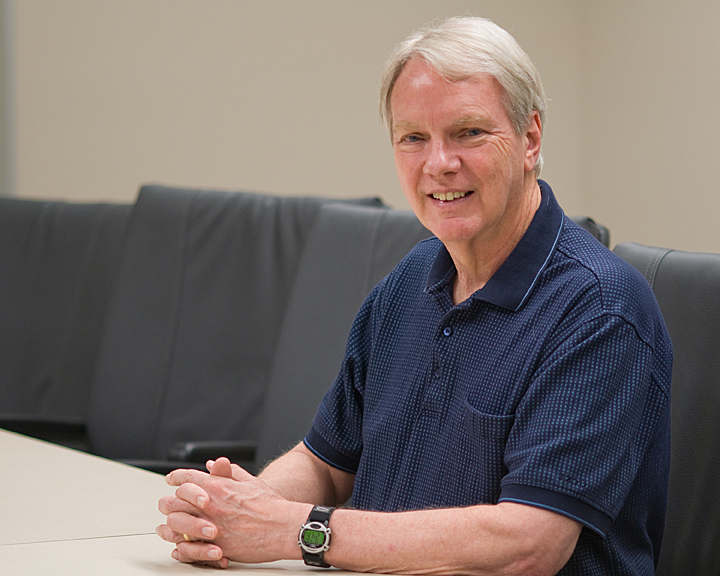In this square image, a Caucasian man in his 60s with short, grayish-white hair, neatly parted on the side, is seated at a light grey table. He has light blue eyes, visible gray eyelashes and eyebrows, and a glowing red complexion. His blue polo shirt, featuring a collar, two buttons, and a visible pocket, boasts a textured fabric with shades of lighter blue. The short sleeves of the shirt extend near his elbows. The man’s face beams with a smile, showcasing his upper teeth and the crinkles around his eyes.

His hands, with fingers interlaced, rest comfortably on the table. Notably, he wears a black watch with a green face on his wrist. There's also a glimpse of a ring on his left hand. Seated on a gray cushioned chair, he faces forward while his body angles slightly to the left. The background showcases a row of similar gray chairs extending to the left, set against a tan or beige wall, blending harmoniously with the tan table he rests upon.